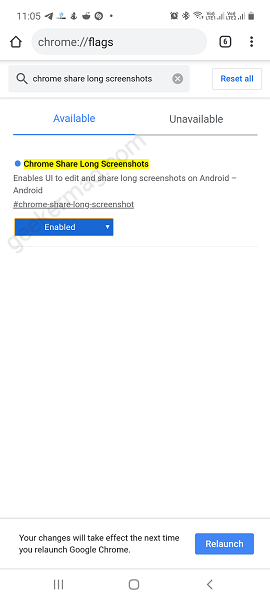The screenshot, captured from someone's smartphone, displays a detailed view of the browser settings page within Google Chrome. The top section of the image includes a white status bar showing the time "11:05", along with icons indicating phone lock status, a Wi-Fi signal with four bars (three of which are filled), and a battery icon. 

Below the status bar is the browser's address bar, which is displayed with a home icon on the left followed by the URL "chrome://flags" in gray text. To the right of the URL are two additional icons: a box containing the number "6" and an icon with three vertical dots.

Under the address bar is a gray search bar labeled "Chrome share log screenshots", with a blue "Reset all" button on its right. Further down, a white section is divided into two tabs: "Available" in blue (highlighted by a blue underline) on the left and "Unavailable" in gray (highlighted by a gray underline) on the right.

The highlighted setting "Chrome share long screenshots" appears next. It is marked with a yellow highlight and reads, "Enables us to edit and share long screenshots on Android". This setting has a corresponding hashtag "#chrome-share-long-screenshot" followed by a blue drop-down menu indicating that the feature is enabled.

At the bottom of the page, a message indicates, "Your changes will take effect the next time you relaunch Google Chrome" accompanied by a blue "Relaunch" button to the right.